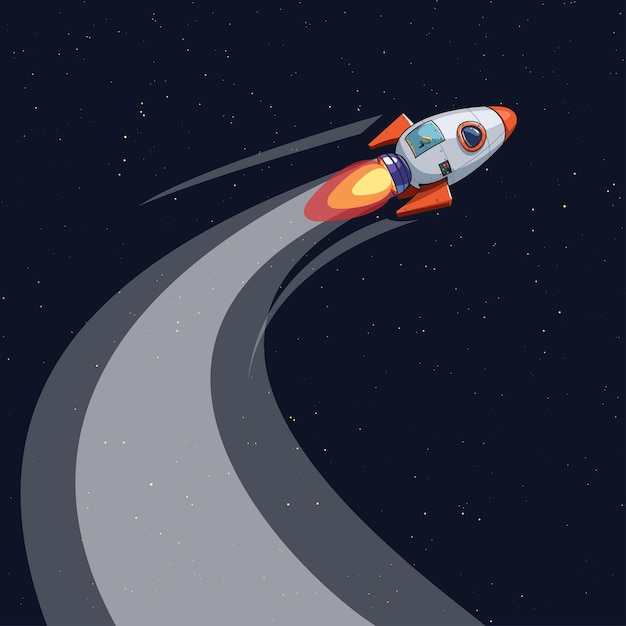This digital graphic resembles a still from a cartoon, depicting an old-style spaceship with an egg-shaped body and a pointed head. The sleek design features two downward angled red fins at the rear. The rocket is primarily gray with vibrant orange accents on its access door, fins, and tip, as well as a circular port window bordered in orange. The engine at the bottom of the ship emits a multi-layered flame with yellow at the core, encircled by orange, and red at the exterior, simulating the varying temperatures of a real flame.

The spaceship is captured as it soars through a dark navy blue sky dotted with white specks representing stars. A dynamic motion trail is illustrated in shades of gray, starting wide from the center left of the image and curving elegantly to the upper right corner, emphasizing the rocket’s swift ascent. Additional smaller motion lines trace the trajectory from the fins, enhancing the sense of rapid movement. The entire scene has a lively, animated quality that suggests the spaceship is journeying through the vastness of space.